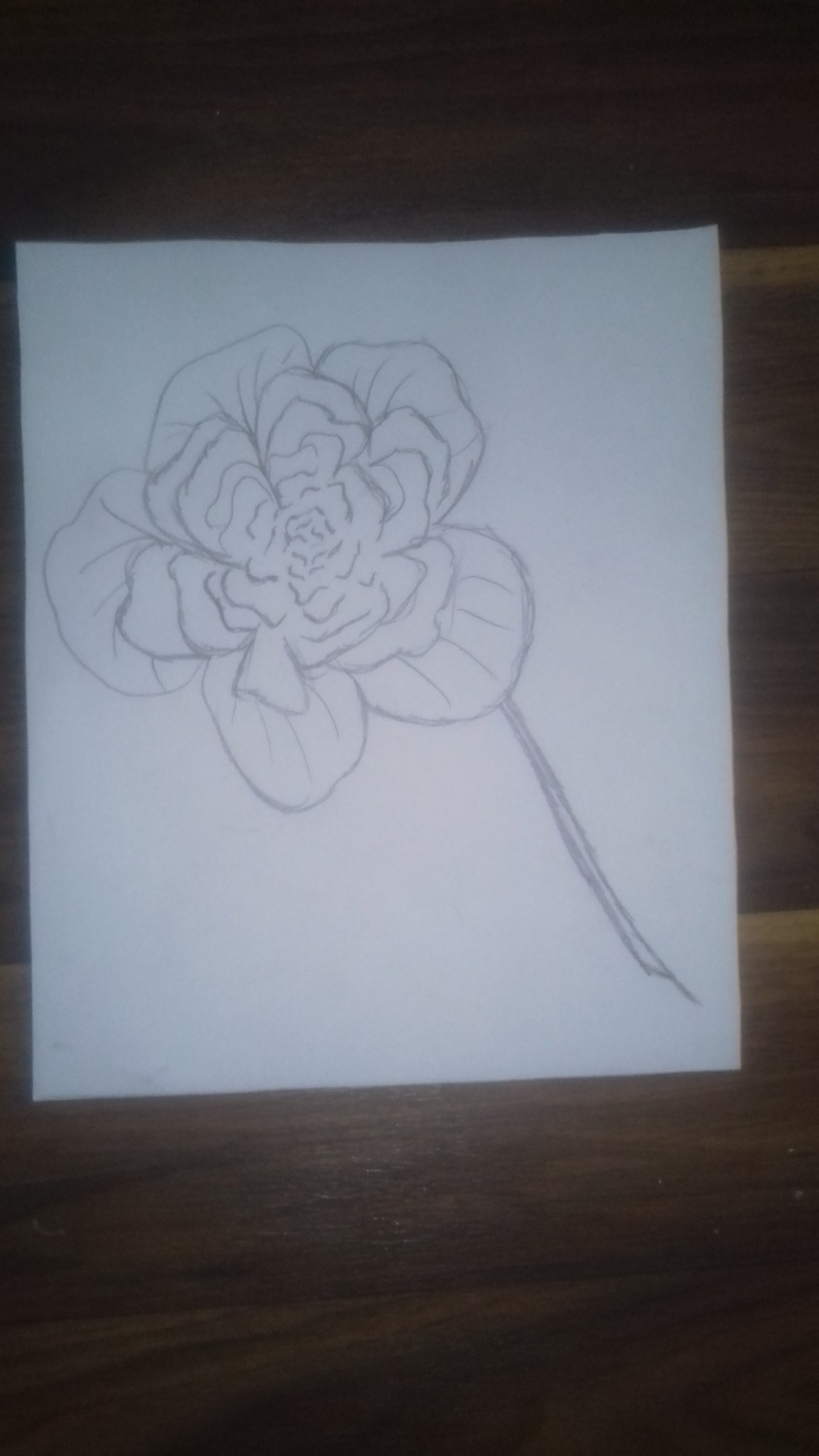A slightly blurry image featuring a rough pencil sketch of an intricate flower on a white piece of paper. The paper rests on a brown wooden surface, likely a table. The flower, yet to be colored or completed, displays an outer ring of five distinct petals surrounding several clusters of inner petals. The stem emerges from the lower right side of the flower, extending nearly to the bottom right corner of the page. Predominantly, the flower occupies the upper left half of the paper, creating a striking yet unfinished depiction of natural beauty.